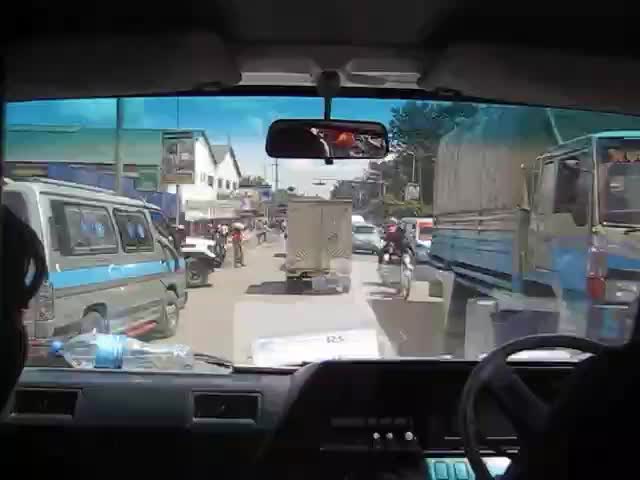This photograph is taken from the inside of a high-seated vehicle, likely a minivan or a similar type, showcasing its large, wide rectangular windshield. Inside, the dashboard, steering wheel, and ventilation system are all gray, with a contrasting white roof. The silhouette of the front passenger's right side of the face and the driver's left shoulder are visible, hinting at their positions.

Outside the vehicle, a busy street scene unfolds, indicating the vehicle is driving on the left side of the road, suggesting locations such as South Africa or India. In front, there's a white mini truck, and to the left, a gray minivan with a cyan-blue stripe down its side, from which the driver's arm is hanging out the window. On the right, a gray and blue truck is passing by, while two lanes of traffic flow in the opposite direction. Additional elements include a person on a motorcycle riding next to a gray truck with a rectangular trailer and a white car visible further left. The street is lined with white buildings on the left and trees on the right, all under an overcast sky. The scene captures the hustle and bustle of a busy urban area during the day.